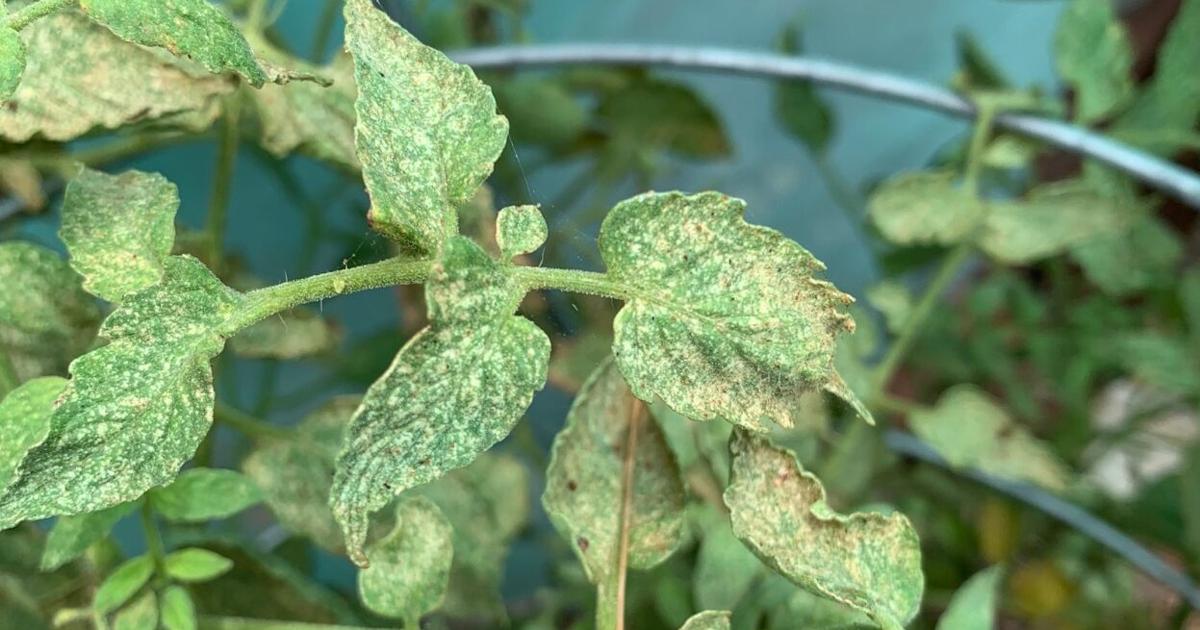This close-up image showcases an outdoor scene featuring diverse plant life set against a blue wall background. Two silver rods stretch horizontally across the frame, providing context and structure. Prominently in the foreground, a vine with a thick, slightly fuzzy stem extends from the middle towards the left side of the image. This vine features multiple leaves, primarily green with some showing signs of distress with brownish and yellowish tinges, while a few exhibit beige freckles, possibly indicating dryness or the onset of recovery. The leaves vary in condition; some appear healthy while others seem crumpled or possibly affected by dust or fungus. Additionally, a portion of a circular metal wreath entwined with the vine is visible. The backdrop includes more green plant life, softly out of focus, enhancing the depth and complexity of the scene.